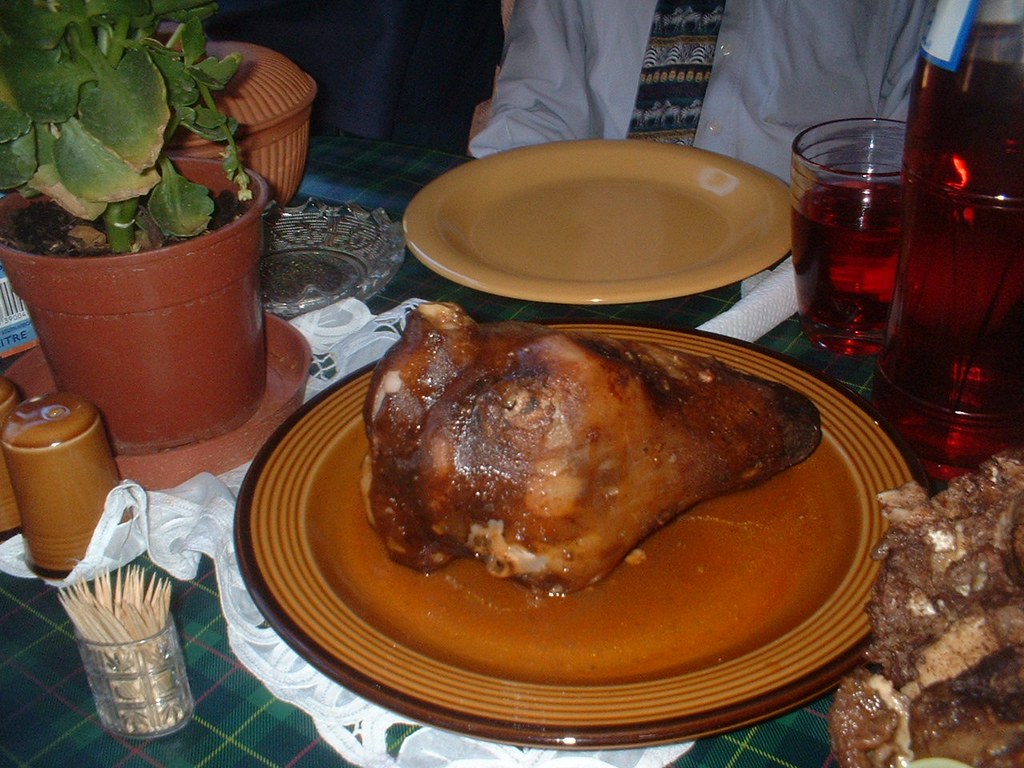This photo, taken indoors at a restaurant, features a detailed table setting that draws the eye immediately to a large, brown-orange plate in the center, showcasing a golden-brown roasted or grilled chicken. This sizable piece of meat dominates the scene and is accompanied by another chunk of meat visible at the bottom right corner of the image. Just behind this centerpiece, a person wearing a white shirt and a quirky tie with zebra patterns can be partially seen, with an empty yellow plate and a glass filled with a brown liquid, likely tea, in front of them. No ice is in the glass. On the right side of this glass, there is a bottle filled with the same brown liquid.

Adjacent to the chicken, there's a potted plant in a brown planter, adding a touch of greenery to the table. Below the plant, a container holding toothpicks is neatly positioned. Also present are what appear to be salt and pepper shakers to the south of the plant. This photo intricately captures the essence of a well-set table ready for a meal, highlighting a large, inviting piece of meat at its heart.